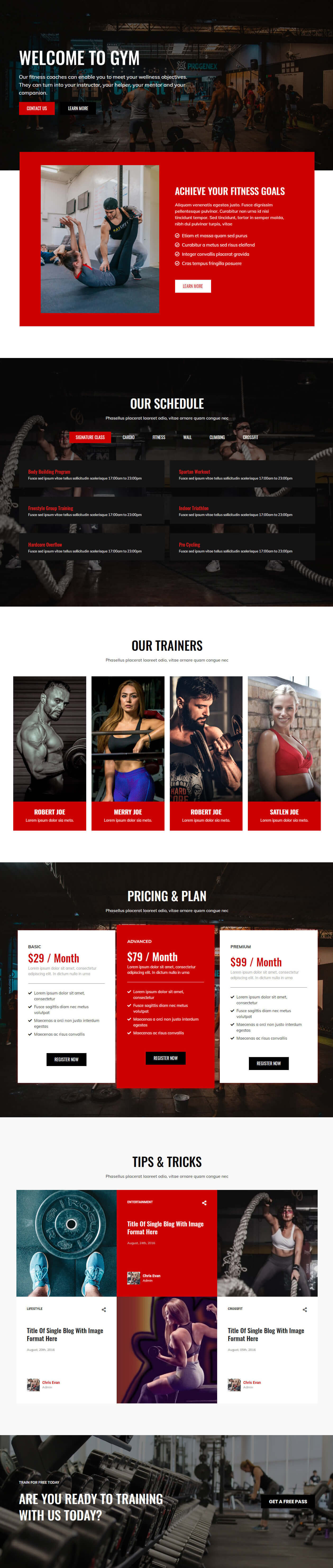The screenshot captures various sections of a comprehensive website dedicated to fitness, presumably named "Jamo." At the very top of the image, in the left corner, there's a small text header that reads "Welcome to Jamo." Though difficult to read in the screenshot, this header is accompanied by a brief welcoming paragraph. Next to this section, on the left side, there's a prominent red button, while the right side hosts additional textual content.

The subsequent section features a headline stating "Achieve your fitness goals," likely acting as an inspirational header. Just below this, there's a segment titled "Our schedule," which appears to list short sentences or phrases, perhaps detailing the fitness programs offered.

Following this, a section labeled "Our trainees" showcases an image of four individuals: two women and two men, potentially members or success stories from the fitness community.

The next segment is designated "Pricing and plan," presenting three different subscription options. The central option specifies a charge of $79 per month, standing out among the choices.

Further down, a section named "Tips and tricks" displays images of individuals working out, with these pictures alternating sides to create a dynamic visual flow.

The final part of the screenshot contains a motivational call-to-action reading, "Are you ready to train with us today?" encouraging immediate engagement from the viewer.